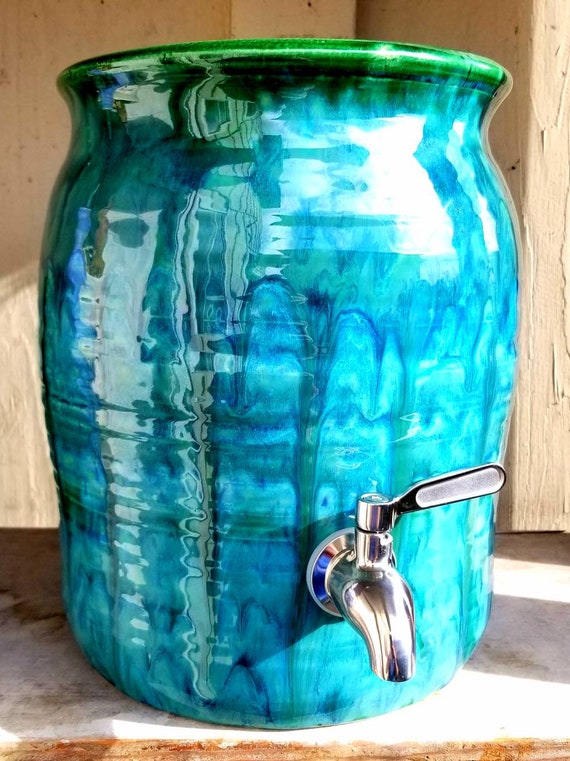The image features a large, ceramic drink container that has been expertly glazed and fired in a kiln. The container showcases a vibrant, streaky paint design that transitions from a rich green at the top to various shades of blue, with noticeable paint drips adding character to its shiny surface. Attached to the bottom of the container is a silver spigot, which is also shiny and equipped with a handle that can be turned to dispense liquids. The canister is situated on a wooden surface, with a wooden background further highlighting its artistic and functional appeal.